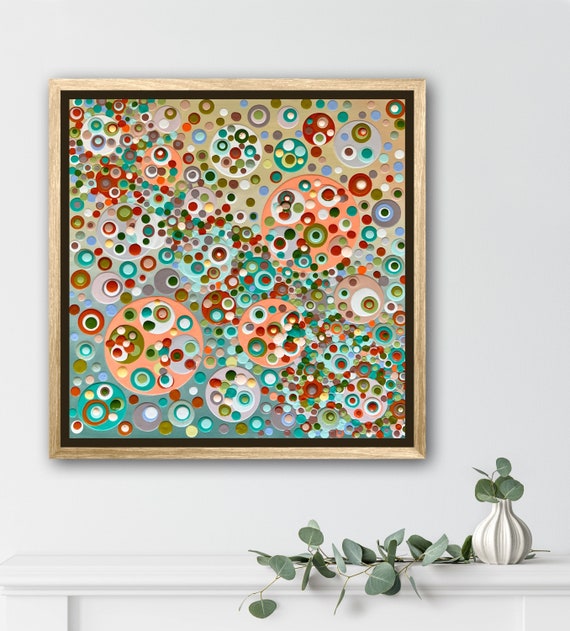The photograph captures a professionally staged indoor setting, ideal for a design magazine. A light gray wall serves as the backdrop, adorned with a vertically rectangular painting encased in a light wooden frame with a black border inside. This artwork features a plethora of overlapping and nested circles in a variety of colors, including red, blue, white, lavender, peach, greens, and turquoises. The larger circles contain numerous smaller circles, creating a visually engaging effect. The painting's background is a subtle beige, with the densest clustering of circles running diagonally from the top left to the bottom right corner. Below the painting, a white mantle runs horizontally, bearing a white onion-shaped ceramic planter from which a delicate green vine, possibly paper, extends and drapes gracefully across the surface. The overall composition is clean and modern, highlighting both the intricate artwork and the minimalist decor.